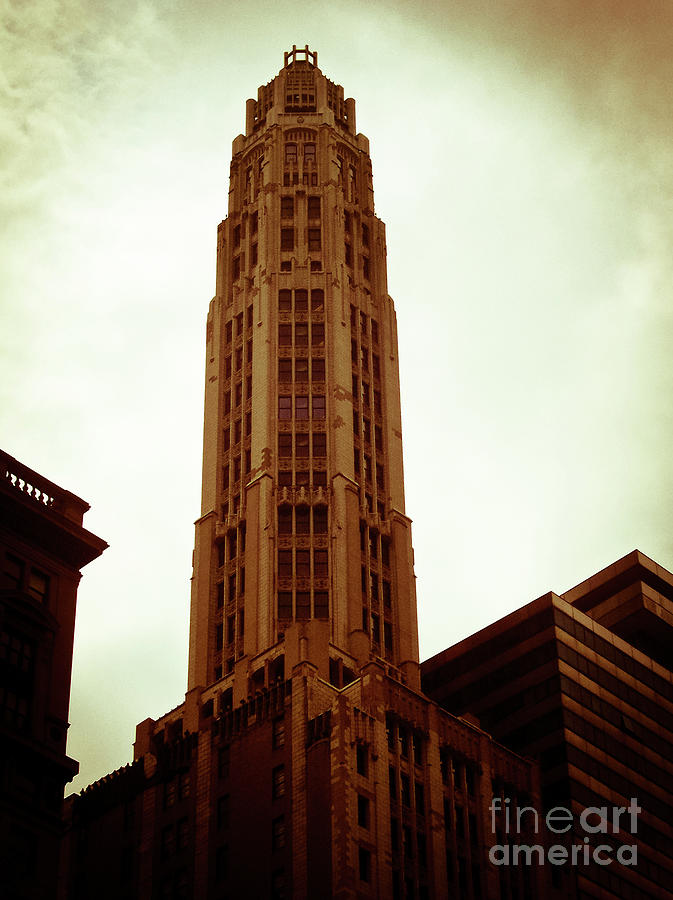The image captures an artistic view of a tall, imposing skyscraper with a unique cylindrical shape, gradually shrinking in segments as it ascends to a peak. The atmosphere is dominated by an apocalyptic, dusky ambiance, with the sky adorned in a blend of grayish yellow and beige tones. This gives the scene a somewhat surreal and dramatic effect. The skyscraper itself exhibits a brownish hue, attributed in part to the coloration of the sky and the play of sunlight. The bottom right corner features a watermark from Fine Art America, with "Fine" in a thinner text while "Art America" is in bold. Adding to the composition, the edges of other rectangular buildings appear in the frame: one intruding from the bottom left and another from the bottom right, providing a contrast to the central structure. Overall, the image evokes a slightly dystopian feel, emphasizing the dramatic aesthetic of urban architecture.